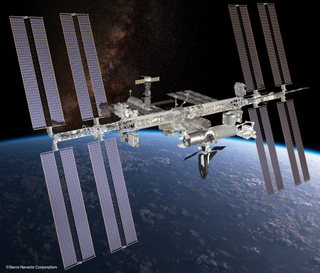In this detailed image captured in outer space, the stark blackness of space dominates the right half of the background. In contrast, the left side features a mystical, white, puffy gas-like material laced with hints of blue, evoking an ethereal sense of the cosmos. Below, the curvature of the Earth is visible, depicted in bold blue hues with intermittent white cloud patterns that seem to bubble up across the planetary surface. Hovering prominently above Earth is a silver-colored satellite, its mechanical structure stark and intricate against the backdrop of space. The satellite's body is adorned with flat, metallic boards or wings that jut out horizontally from both the top and bottom sides. Each wing ends in what appear to be solar panels or blades, arranged in pairs, making a total of four on each side. Hanging centrally from the satellite are small camera-like devices. The contrast of the technical, silver, gray, and black components of the satellite with the vibrant blue Earth and the dark void of space creates a visually compelling scene, showcasing the blend of human ingenuity and the vastness of the universe.